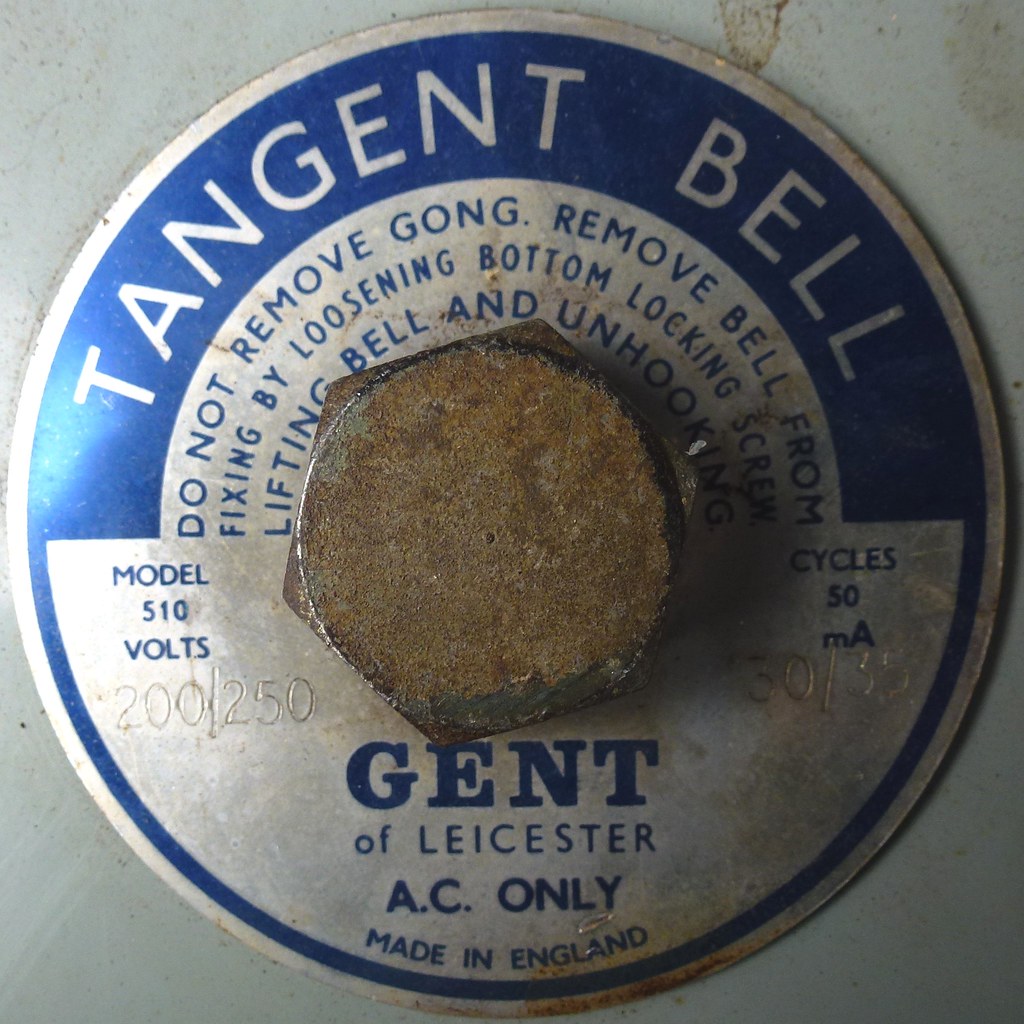The image is a square photograph prominently featuring an old, rusted, metallic surface. Centered in the forefront is a large, rusty hexagonal bolt securing an informational circular tag to the surface. The tag predominantly displays a color palette of blue, white, and a touch of silver, brown, copper, and gray, contributing to the aged appearance of the setting. 

At the very top half of the tag, there is a distinctive blue banner with the white text "Tangent Bell". Directly beneath the banner is a cautionary note in blue text stating, "Do not remove gong. Remove bell from fixing by loosening bottom locking screw, lifting bell, and unhooking." On the left side of the tag, the text reads "Model 510 Volts," and on the right side, it specifies "Cycles 50 MA". Additional information is inscribed at the very bottom: "Gent of Leicester AC only. Made in England." Contributing to the authenticity and age, the tag also features punched numbers "200/250".

The meticulously detailed elements and textual instructions on the tag suggest its purpose as a functional component, likely related to an old bell or gong mechanism, although the exact function remains ambiguous.